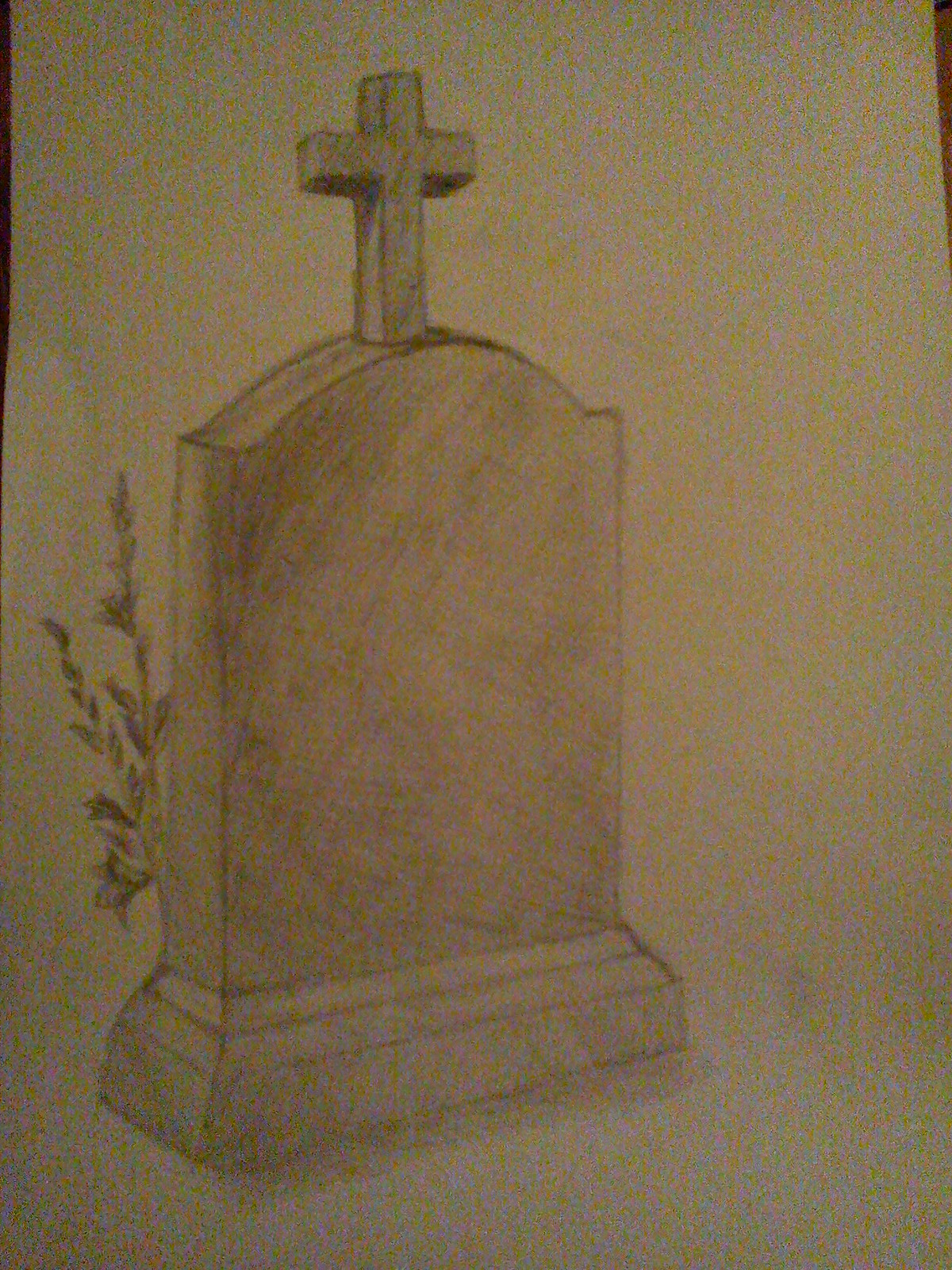A meticulously sketched 3D coffin is presented, seemingly drawn on a piece of paper that shows faint shrivels at the top, suggesting it is laid on a table. The attention to detail in this artwork is extraordinary, with the 3D depiction of the coffin making it appear strikingly lifelike, akin to a prop from a movie. The drawing medium appears to be pencil or charcoal, contributing to the deep, rich hues and precise lines that give the coffin its realistic appearance. The coffin, designed with a rectangular base that slightly narrows upwards, features an intricately rendered 3D cross on its lid. Surrounding the coffin, faint sketches of flowers or bushes are discernible—depicted with hints of green and purple—adding subtle color and texture to the background. These floral elements are situated to the left side of the coffin, enhancing the scene's depth. The lower part of the coffin displays a set of three finely drawn lines, further emphasizing the artist's skill in capturing intricate details. A soft shadow beneath the coffin suggests daylight illumination, enriching the dimensionality of the artwork. The piece lacks any inscribed names, focusing instead on the cross as the central emblem on the coffin lid.